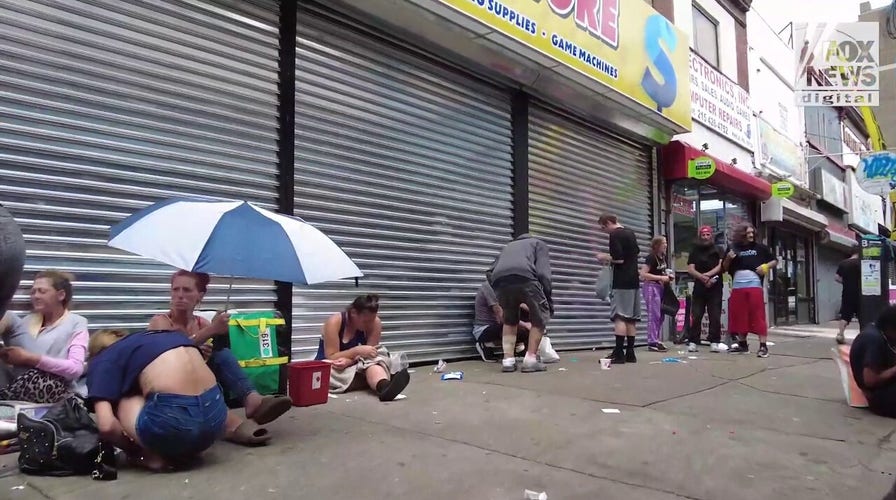The image depicts a city sidewalk in front of a closed store with a prominent yellow awning, secured by a large silver gate segmented into three sections by black vertical poles. Several homeless individuals are scattered along the pavement. At the left side of the image, a woman is sitting on the ground holding a blue and white umbrella. In the foreground, another woman squats with her tote bag next to her, while nearby, a barefoot woman with sandals rests next to her belongings. Trash and debris litter the sidewalk, emphasizing a state of neglect. In the background, a sign reading "Fox News Digital" is noticeable, and several individuals are either standing or sitting in groups, engaging in conversations. Some people are standing alone facing the storefronts, which remain closed. The individuals are dressed casually, wearing items like long shorts and t-shirts.